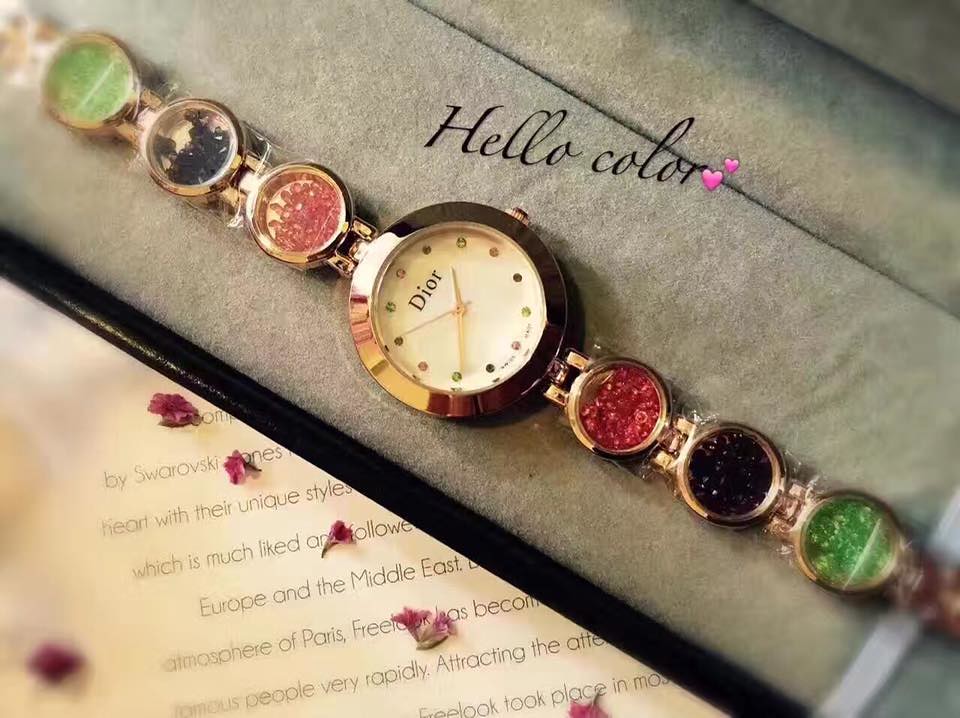This advertisement image for a Dior watch showcases the elegance of the timepiece with immaculate detail and luxurious presentation. The watch is displayed at an angle running from the top left to the bottom right corner, nestled atop a gray felt cushion within a black box. The watch features a distinctive design with a central time-telling circle, complemented by an artistic arrangement of variously colored circles forming the band. The main watch face, larger than the surrounding circles, is a pristine white adorned with abstract circle markers for each hour, and gold hour and minute hands. The brand name "Dior" is prominently displayed below the 12 o'clock position in sleek black text. 

Surrounding the central circle are additional circles filled with vibrant stones—an array featuring light pink, dark pink, black, and various shades of green, giving a dynamic yet harmonious aesthetic to the watch.

Above and to the right of the watch, the phrase "HELLO COLOR" is engraved in black on the gray felt, accompanied by two small pink hearts near the "R." This message sits in sync with the watch's colorful design, echoing a playful yet sophisticated vibe. Below the box lies a white piece of paper covered in partially visible black text and scattered with delicate flower petals, adding a soft, romantic touch to the scene. The overall image is presented with a focused center and blurred edges, drawing the viewer's attention straight to the luxurious watch and its splendid details.